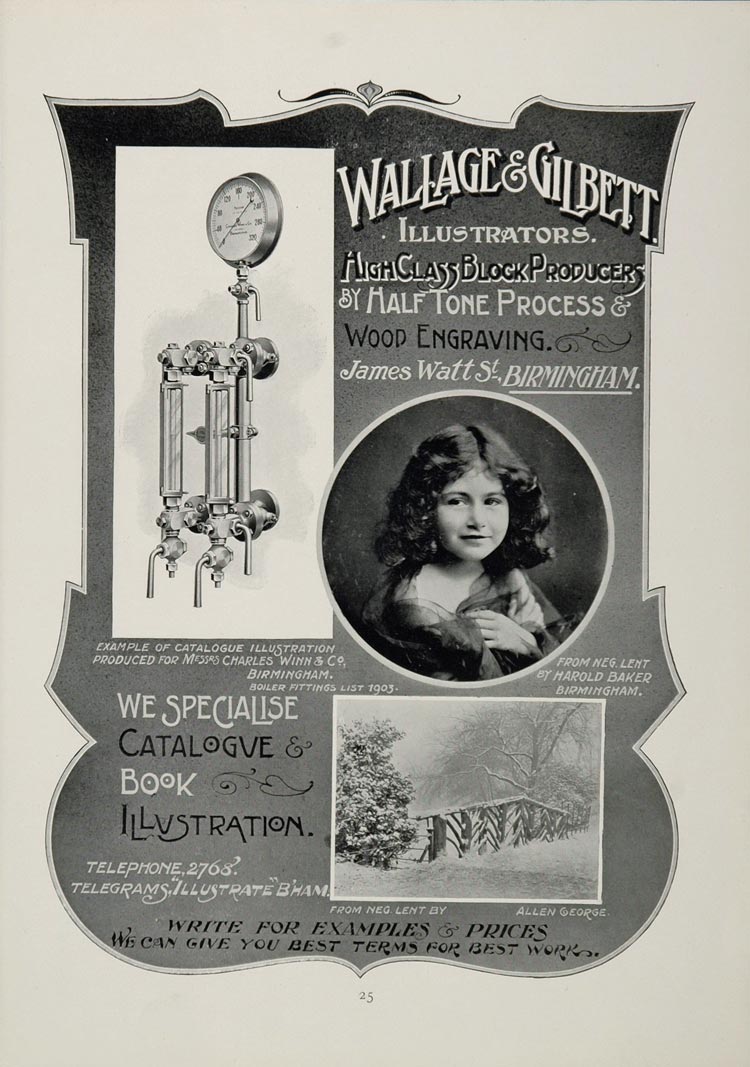This vintage advertisement, shaped like a shield, represents Wallage and Gilbert, illustrators known as high-class block producers specializing in halftone processes and wood engraving. The poster prominently displays their slogan "High Class Block Producers, by Halftone Process and Wood Engraving." The top of the ad reads "Wallage and Gilbert, illustrators," followed by their address, "James Watt St., Birmingham."

At the center of the advertisement is a circular, black-and-white photo of a young girl with dark, curly hair, gazing to the left. To the left of her image is a hand-drawn illustration of a pipe with a gauge. Below the girl’s image, additional hand-drawn artwork depicts a snowy bridge scene. In the lower-left corner, the text mentions their specialization in catalog and book illustrations, along with the note: "We specialize catalogs, books, and illustrations. Telephone 2768, Telegraph Illustrate." At the bottom of the poster, the text encourages potential clients to "write for examples, prices. We can give you best terms for best work."